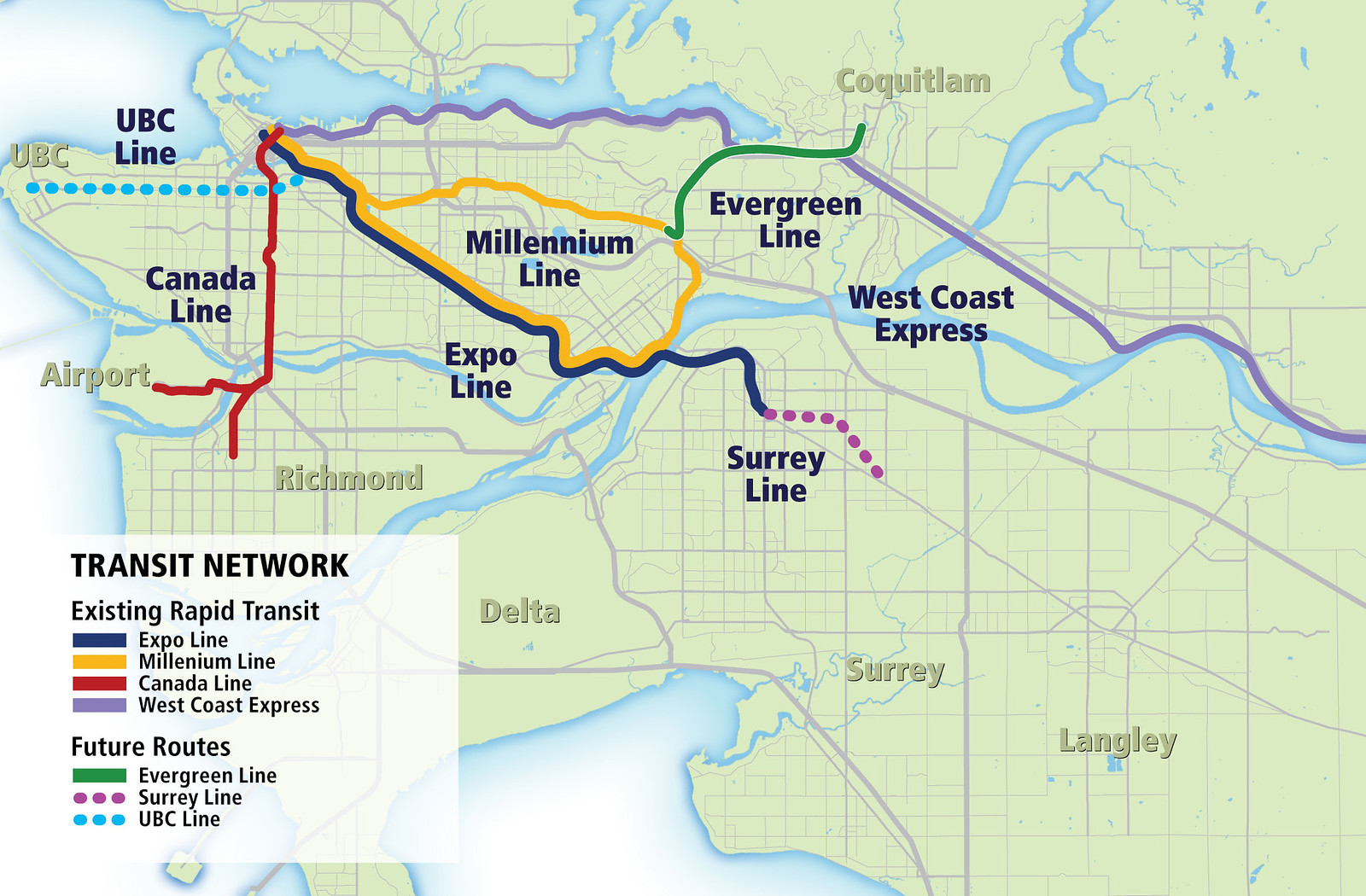This image depicts a digitally drawn map of a transit network, primarily in pale green to represent land and blue for bodies of water, including rivers, channels, and the ocean. The map, which covers the entire picture except for a white legend box located in the lower left-hand corner, showcases various rapid transit lines such as the Expo Line (navy blue), Millennium Line (yellow), Canada Line (red), West Coast Express (purple), and the Evergreen Line (green). Additionally, it indicates future routes like the Surrey Line (purple dots) and UBC Line (blue dots). The legend clearly categorizes the different transit lines under "Transit Network," distinguishing between existing lines and future routes. Surrounding cities like Richmond, Delta, Surrey, and Langley are also marked, adding context to the region covered by the transit lines.